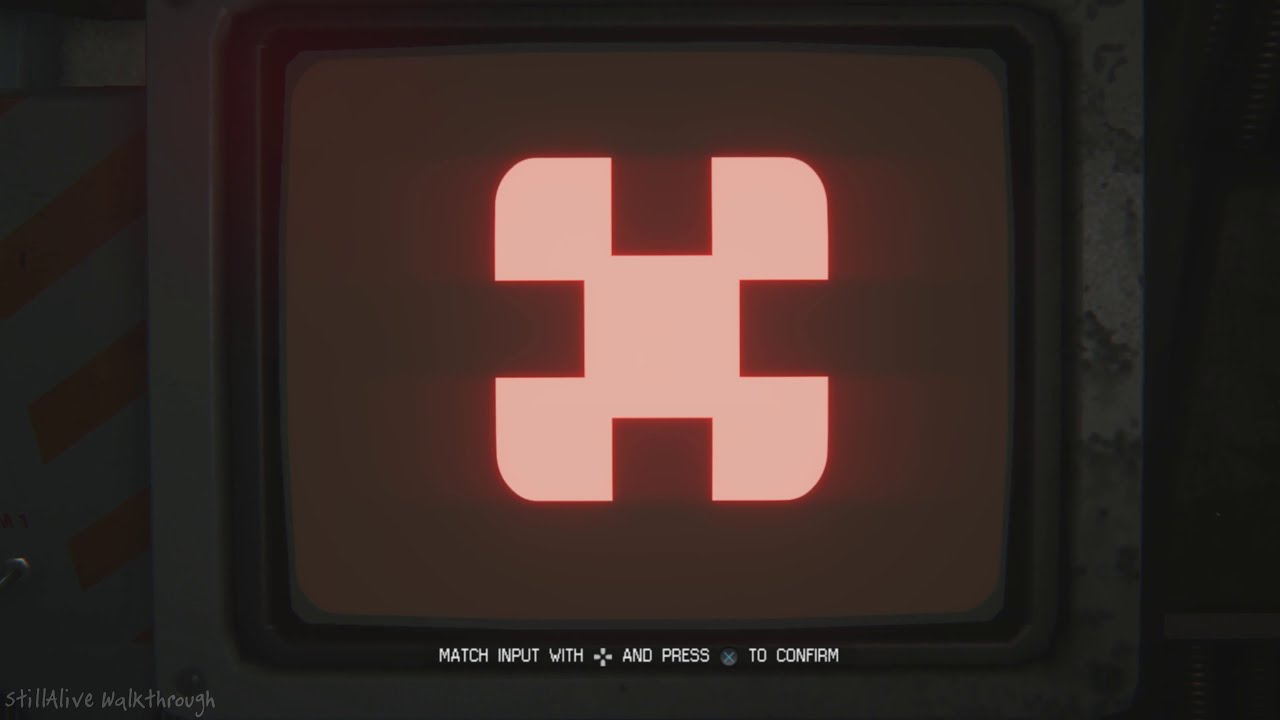This image portrays an old, somewhat blurry television screen featuring an in-game screenshot from a rudimentary video game. The screen, a standout with sharp focus relative to the background, prominently displays a message in white text: "Match input with" followed by a button symbol, and "Press the X button to confirm." The X button is depicted in blue, commonly associated with PlayStation controllers from PS1 through PS5. The game interface, part of a puzzle game, shows squares and a glowing orange element or figure that some described as windmill-like. The surrounding television frame is gray, and the lower corners of the screen feature light white handwritten text reading "still alive, walk through." The background on either side of the screen appears blurred and indistinct.